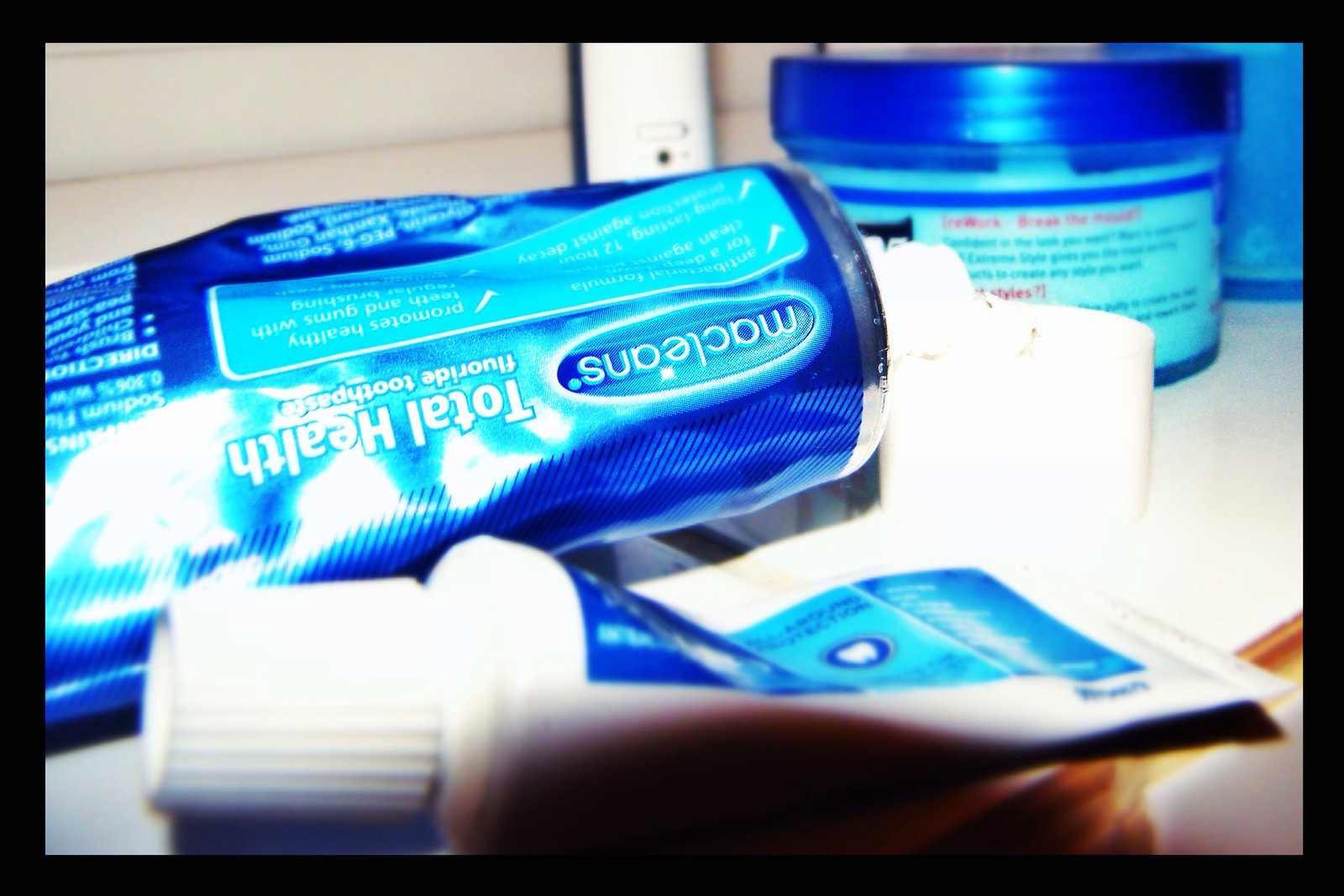This is a detailed close-up image of three personal care items against a white background with a black trim. The primary focus is a partially squeezed blue tube of McLean's Total Health Fluoride Toothpaste, prominently displaying white text despite being upside down. This toothpaste has a distinct white cap lying separately on the white counter. In front of this large tube is a smaller, similarly colored travel-sized toothpaste tube, also squeezed in the middle with a blue label and white cap. To the right is a small jar with a blue lid, featuring a blue label adorned with both dark blue and red writing, though the text is illegible. The background appears to be white and possibly features vertical or horizontal blinds, adding to the clean aesthetic of the image.